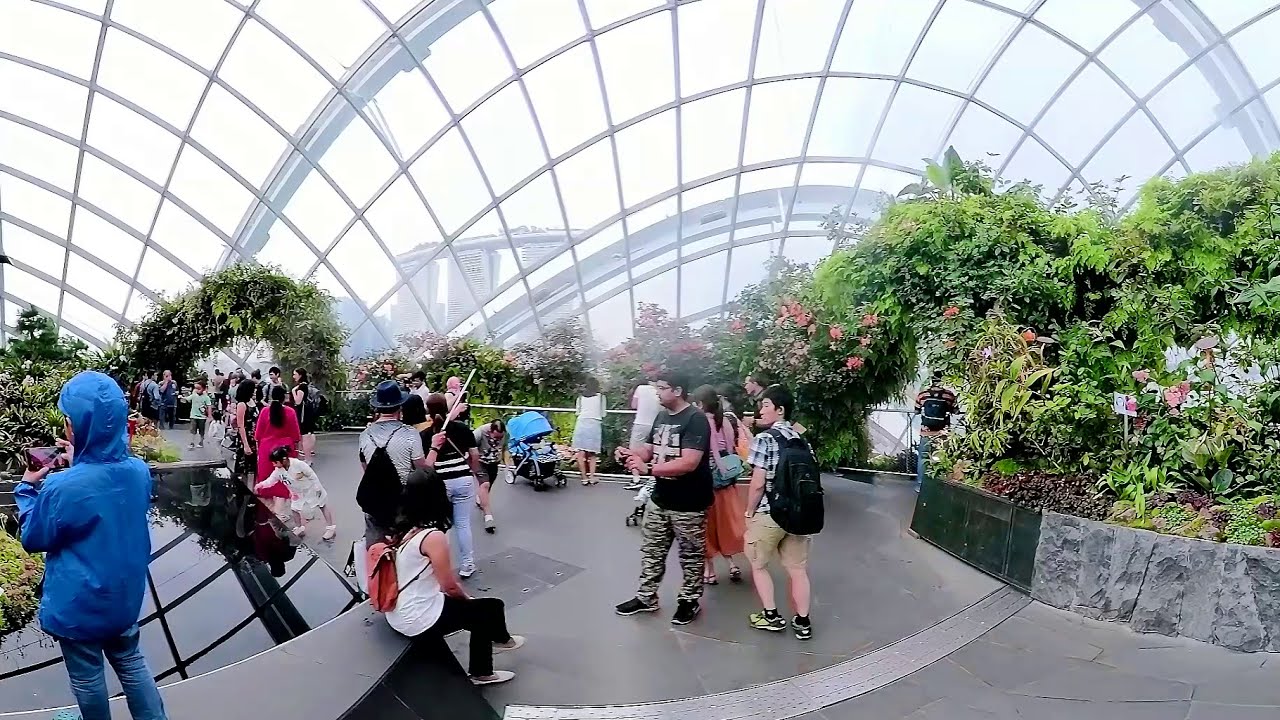The image depicts a bustling indoor garden with a domed glass ceiling, segmented by metal bars, that allows ample sunlight to illuminate the scene. The garden features lush, meticulously maintained foliage, including ivy, flowers, and various other plants growing on rock walls lining a central walkway. The atmosphere is lively, with numerous people strolling, talking, and observing the verdant surroundings. A woman is seen taking pictures of plants on the left side, while others, including a man holding a stick and someone pushing a baby carrier, navigate the crowded walkway. Some children are present, suggesting the possibility of a field trip. The area appears designed as a tourist attraction, possibly within a greenhouse or zoo, where the controlled environment ensures optimal conditions for the indoor greenery. In the bottom left, a person in a blue hooded jacket and jeans stands, while nearby, a person with a red backpack sits on a bench. In the center, a man in camo pants and a black t-shirt with short dark hair is present. The entire scene is set against a backdrop of distant buildings and a bright sky visible through the transparent, temperature-regulating roof.